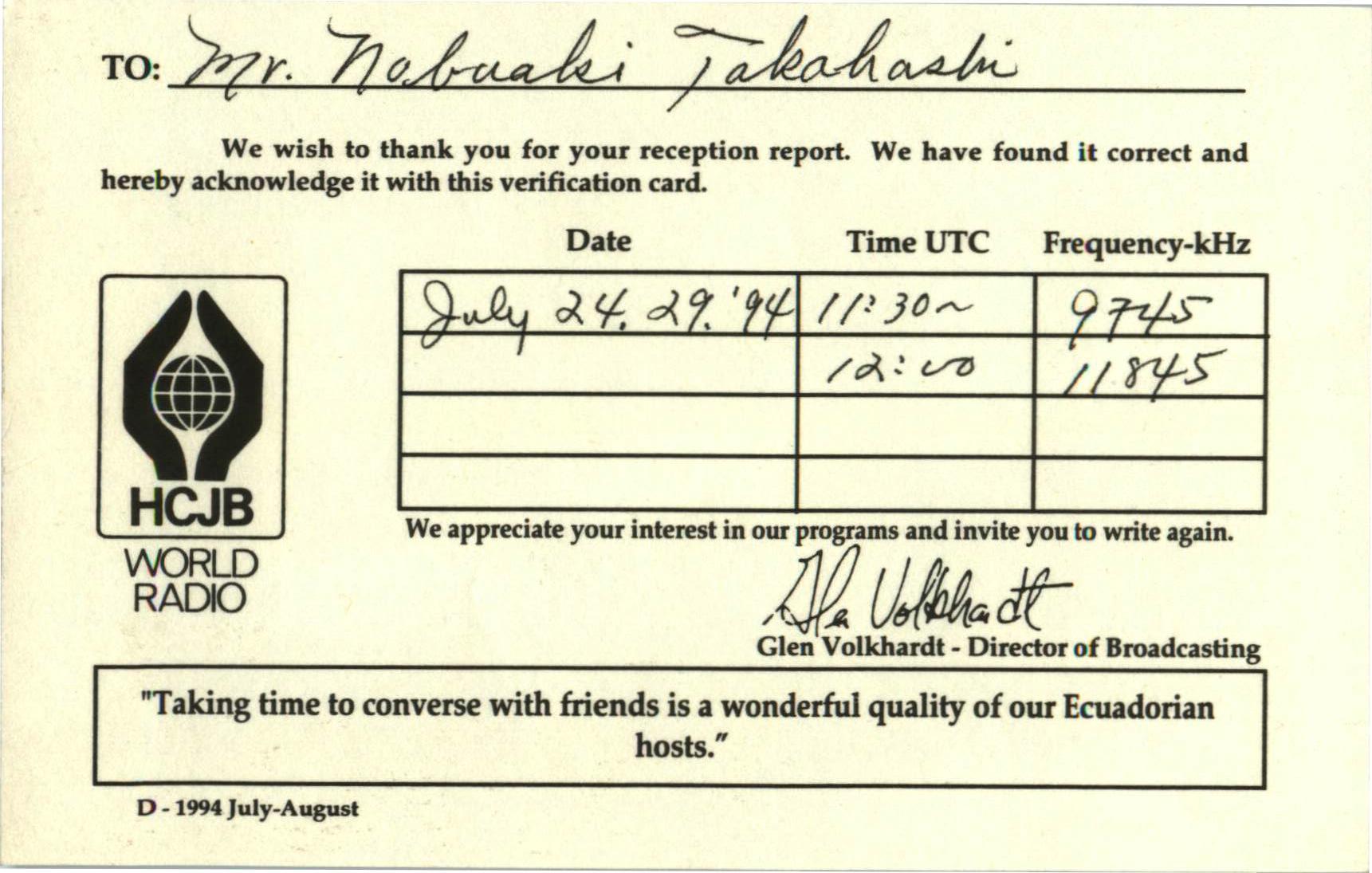The image depicts a verification card with a yellow hue, possibly appearing slightly pinkish. At the top left, it reads "To: Mr. Nobelski Tabaloski" in cursive, followed by a black line. Directly below, in black text, the card expresses gratitude for a reception report, stating, "We wish to thank you for your reception report. We found it correct and hereby acknowledge it with this verification card."

On the bottom left of the card, there's an emblem showing a pair of hands cradling a globe, captioned "HCJB World Radio." Adjacent to this emblem is a chart with columns labeled "Date," "Time," and "Frequency, kilohertz." The entries are handwritten as follows: Date - July 24, '94; Time - 11:30 and 12:00; Frequency - 9745 and 11845 kHz. Below this chart, a note reads, "We appreciate your interest in our programs and invite you to write again."

Further down, the card is signed by Glenn Volkhart, identified as the Director of Broadcasting. A notable quote is featured at the bottom: “Taking time to converse with friends is a wonderful holiday for our Ecuadorian hosts.” In the bottom left corner, it is dated as "D-1994 July-August."